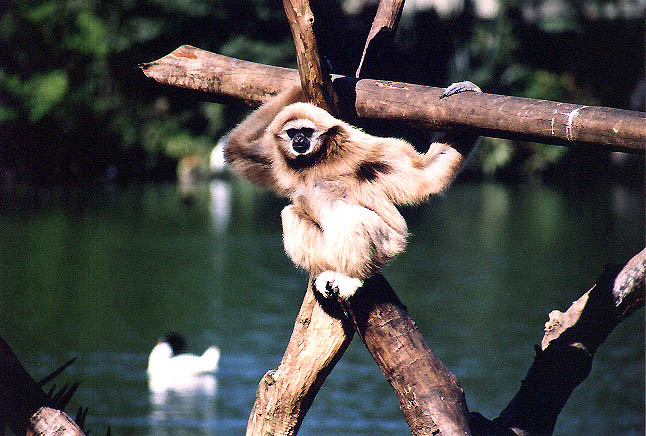This image captures a white-cheeked gibbon, a smaller and furrier species of monkey, characterized by its golden, tan, and white fur and distinctive black face bordered by white. The gibbon is posing against a background of blurred green foliage, indicating a forest, with a body of water (possibly a lake or stream) visible. A white figure, likely a duck or swan, floats on the water in the bottom left corner. The gibbon is perched on a rustic wooden fence made of logs forming an 'X' at the base. Its one arm, darker brown, and the other arm, lighter in color, are wrapped around the central post of the fence. Its feet rest on a smaller branch below. The gibbon's position, with its back to the fence and stomach facing forward, creates an engaging and dynamic composition focused solely on the monkey.